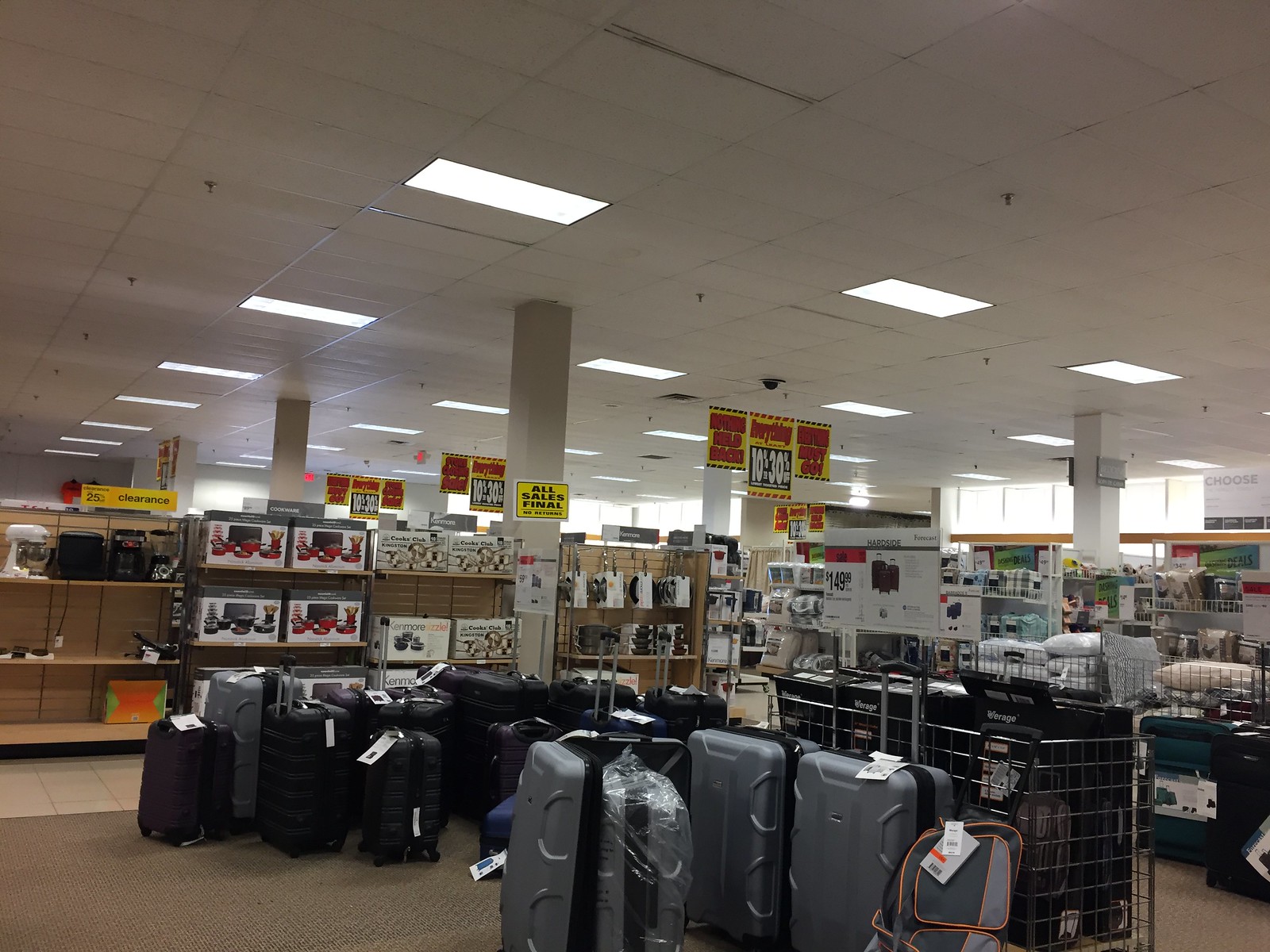A bustling luggage section in a large department store reveals an assortment of gray and black suitcases scattered on a carpeted floor. A sizable metallic bin in the foreground overflows with smaller luggage pieces, hinting at a variety of styles and sizes. Just behind the bin, several containers are stocked with pillows, offering a diverse selection. An aisle separates this section from another area populated with kitchenware. Across the aisle, shelves display a mix of boxed items, including blenders and mixers, while a row of assorted kitchen utensils hangs neatly from a pegboard. The space is illuminated by fluorescent lighting, and numerous signs dangle from the ceiling, guiding shoppers through the expansive store. Additional shelves filled with various products can be seen extending into the background, adding to the cavernous feel of the retail setting.